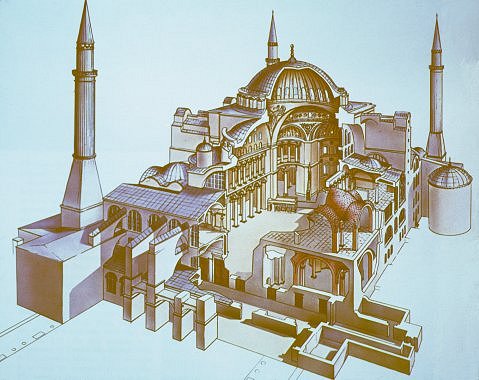This is a detailed artist's rendering of a grand architectural structure, potentially a Roman temple or a cathedral, drawn in a three-quarter view with a meticulous cutaway to reveal the interior. The structure spans approximately one city block and varies in height from two stories in the front to three or four stories toward the rear. Dominated by a multitude of architectural forms, the edifice boasts flat, slanted, and prominent domed roofs, with the rear dome standing out as a key feature.

The cutaway invites viewers to explore the interior, where we observe an array of vaulted arches and multiple levels of columns, including two tiers of columns on the left side. The structure's walls and roofs appear to be constructed from stone, consistent with Roman design elements. The exterior features pointed structures resembling rockets at the front left corner, back corner, and back right corner, accompanied by a cylindrical shape with a small domed top situated in front of the back right pointed structure.

The artwork is rendered in a monochromatic palette of whites, grays, and shadows, creating a minimalistic yet intricate depiction. The detail extends to the floor plan, revealing hallways, pillars, and a grand entrance supported by pillars, enhancing the sense of architectural grandeur.